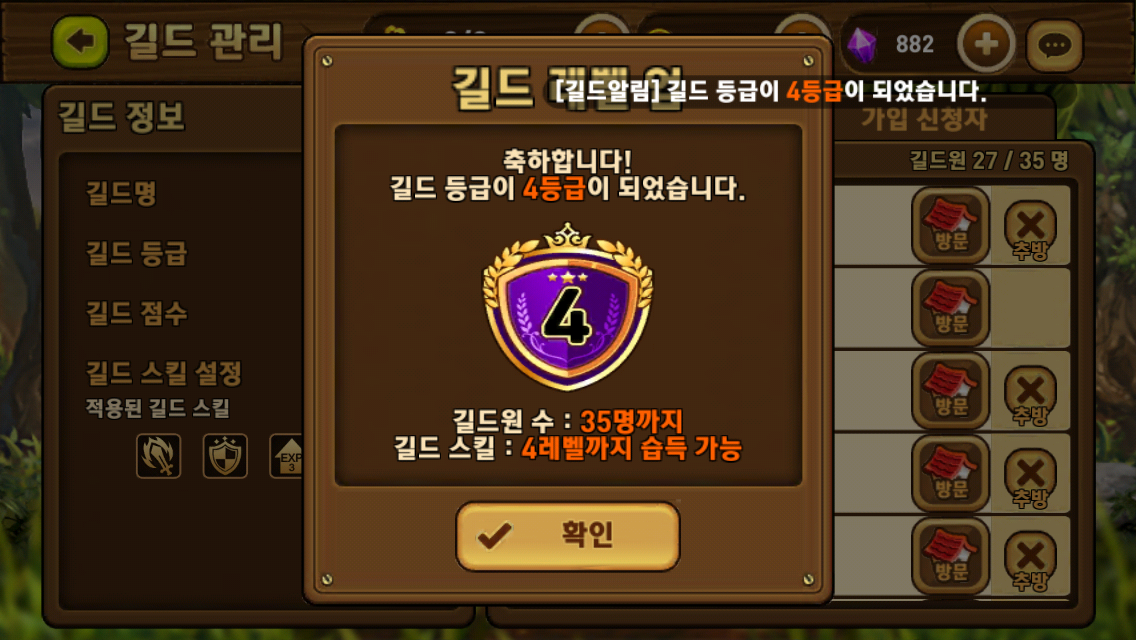This image is a detailed screenshot from the Korean video game "Cookie Run." The interface is predominantly brown with an outdoorsy, woody theme. The top of the screen features important in-game currencies such as gold points and purple diamonds, with a tally displayed in Korean numerals. Central to the image is a large, ornate, wooden-framed square with bolts in each corner, resembling a plaque or trophy. In the middle of this frame, there is a purple shield-like emblem with a gold trim and a prominent black number "4," indicating the player's current level or ranking. Surrounding this central square are various interface buttons, including a white back button with a brown arrow in the upper left corner and additional functional buttons distributed across the screen. In the bottom section, there's a brown clickable button for further actions. On the right side of the screen, there is a list likely indicating player rankings or levels, distinguished by small icons like a house with a red roof and symbols such as X's, with one row notably lacking an X. The entirety of the text and numbers is in Korean, emphasizing the game's origin and the player's level progression.